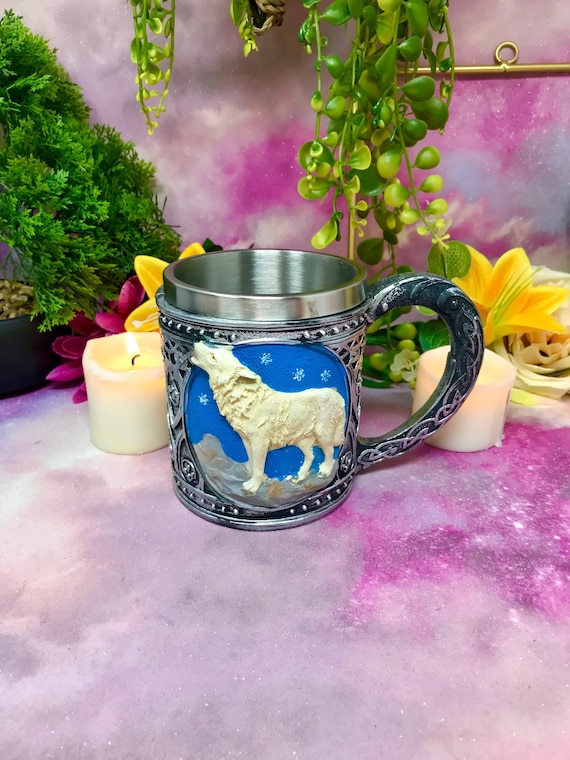The image showcases a detailed and aesthetically pleasing display set on a surface that resembles white granite with bright pink crystals, extending into the backsplash. Central to the image is a silver, stainless steel mug with a large, carved handle. The body of the mug features intricate artwork depicting a howling white wolf set against a blue sky adorned with snowflakes. This circular artwork also shows a greyish landscape at the bottom. The mug sits squarely in focus, drawing attention to its reflective, polished surface.

Flanking the mug are two small votive candles, with the candle on the left clearly lit. The background complements the display with a gradient of pink and magenta hues, both on the wall and the surface. Overhead, green succulent plants drape down, resembling creeping vines, and a pine-like branch adds a touch of evergreen. Yellow iris blossoms and scattered pink daisy petals add further floral elements to the scene. The combined effect of these elements creates a rich, multi-textured backdrop that enhances the central focus of the silver mug and its detailed artwork.